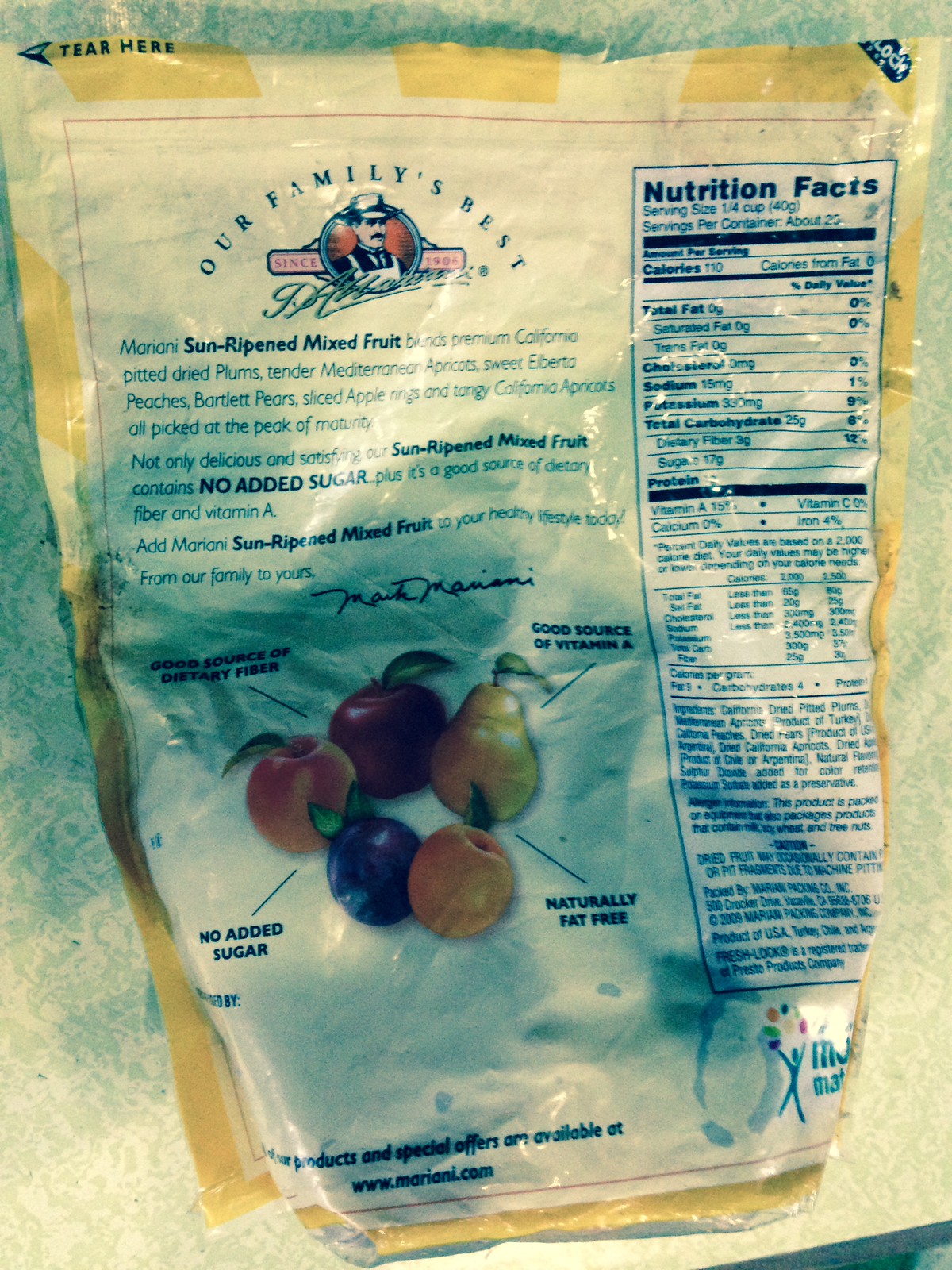On a rustic wooden surface marred with various markings, there lies a plastic bag prominently featuring the label "Our Family's Best." The bag showcases a red circle enclosing an image of a cheerful figure with a mustache, wearing a white apron and a wide-brimmed hat suggestive of a farmer or cowboy. 

To the right of the image, the bag details nutritional information, stating: "Nutrition Facts," with specifics such as "Serving Size: 1/4 cup," and categories including "Calories: 1xx," "Total Fat: 0g," and "Cholesterol: xxmg," followed by more nutritional data in smaller text. 

On the left side of the bag, text reads: "Marianne's Sun-Ripened Mixed Fruit, Premium Dried Plums, Tender Mediterranean Apricots, Sweet Alberta Peaches, Bradley Pears, Sliced Apples, Tangy California Apricots." Below this, a promotional message highlights: "Not only delicious, that's why our Sun-Ripened Mixed Fruit contains no added sugar, plus it's a good source of dietary fiber and vitamin A. Add Marianne's Sun-Ripened Mixed Fruit to your healthy lifestyle today, from our family to yours." There are also illustrations of apples, plums, and pears, along with claims like "Naturally Fat-Free," "No Added Sugar," and other descriptive text.